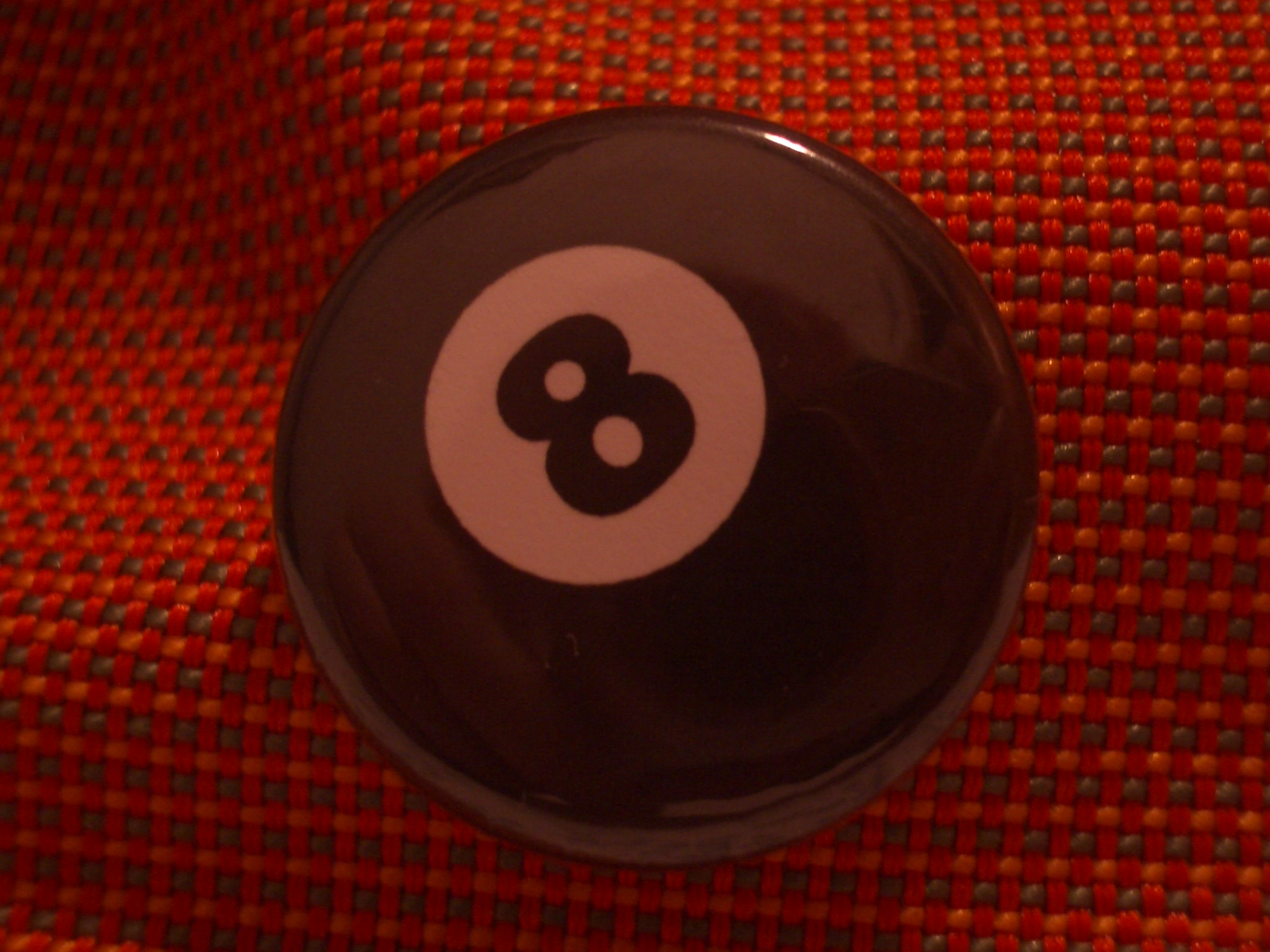This detailed landscape-format color photograph features a close-up of a glossy black 8-ball, prominently showcasing its iconic white circle with the thick number 8. The ball appears to be highly reflective, capturing vague reflections that could involve the photographer, though the specifics remain indistinct. The 8-ball is perched atop an undulating woven fabric, which seems folded in areas, contributing to its textured and wavy appearance. The intricate design of the fabric incorporates a mix of interwoven colors, including orange, red, brown, green, and yellow, creating a visually rich background. Light shines from the top left of the frame, casting discernible shadows and enhancing the three-dimensional feel of both the fabric and the ball. The overall composition is simple yet detailed, focusing on the contrasting smoothness of the 8-ball against the complex patterns and textures beneath it.